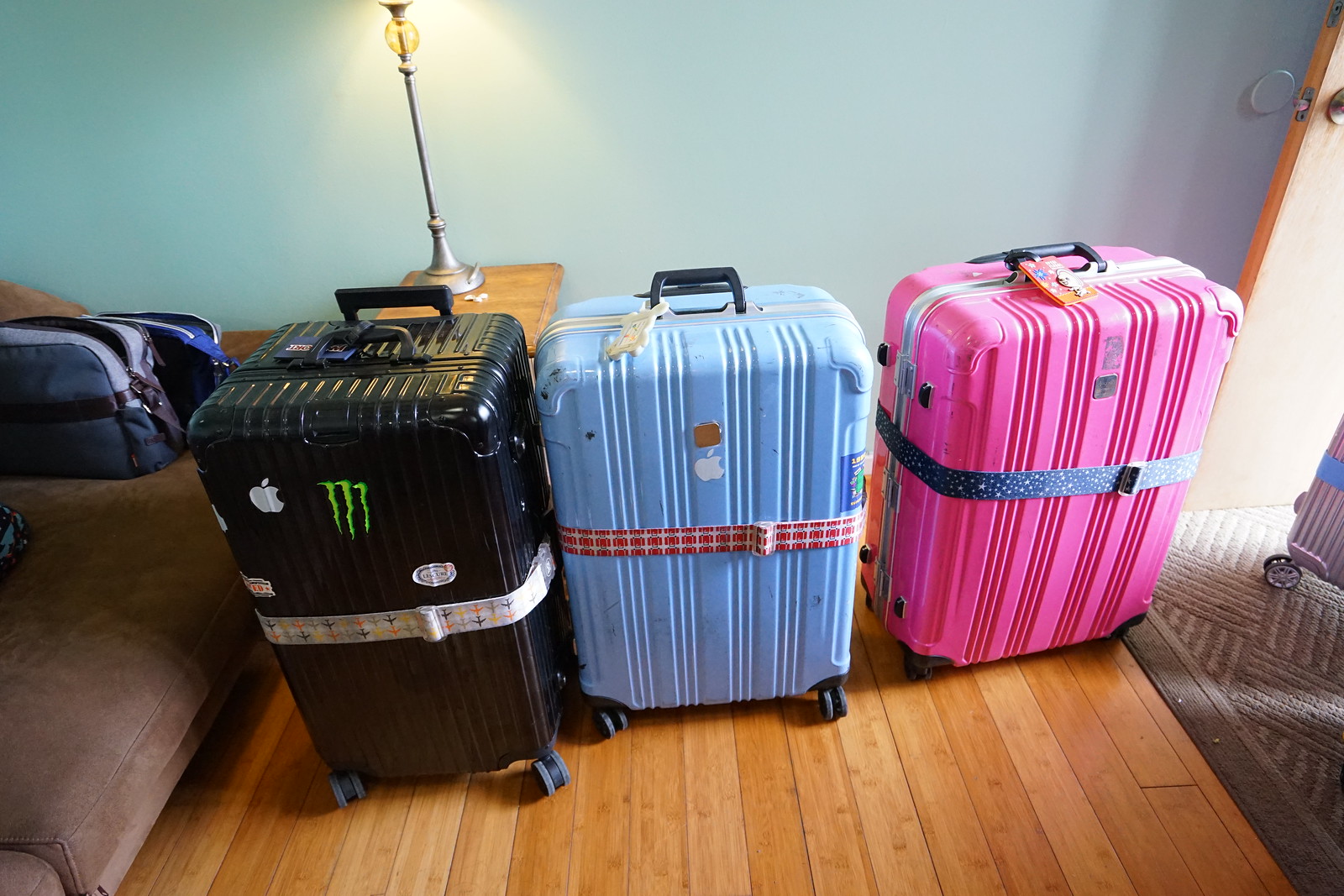In this color photograph, three hard-shell, upright carry-on suitcases on wheels are prominently displayed against a light wood laminate floor. The suitcase on the left is black with visible Apple and Monster Energy Drink logos and a white belt around it. The middle suitcase is a light sky blue, also featuring an Apple logo and secured by a white and red strap. The suitcase on the right is hot pink with a black strap that includes a white design. These suitcases are all standing upright. To the left of the scene, a brownish-beige couch is visible, adorned with a couple of duffel bags in various shades of blue. The backdrop includes a blue wall with a wooden tabletop and the lower part and neck of a lamp, casting light downward. An open door and part of a carpet are also visible on the right side of the image.